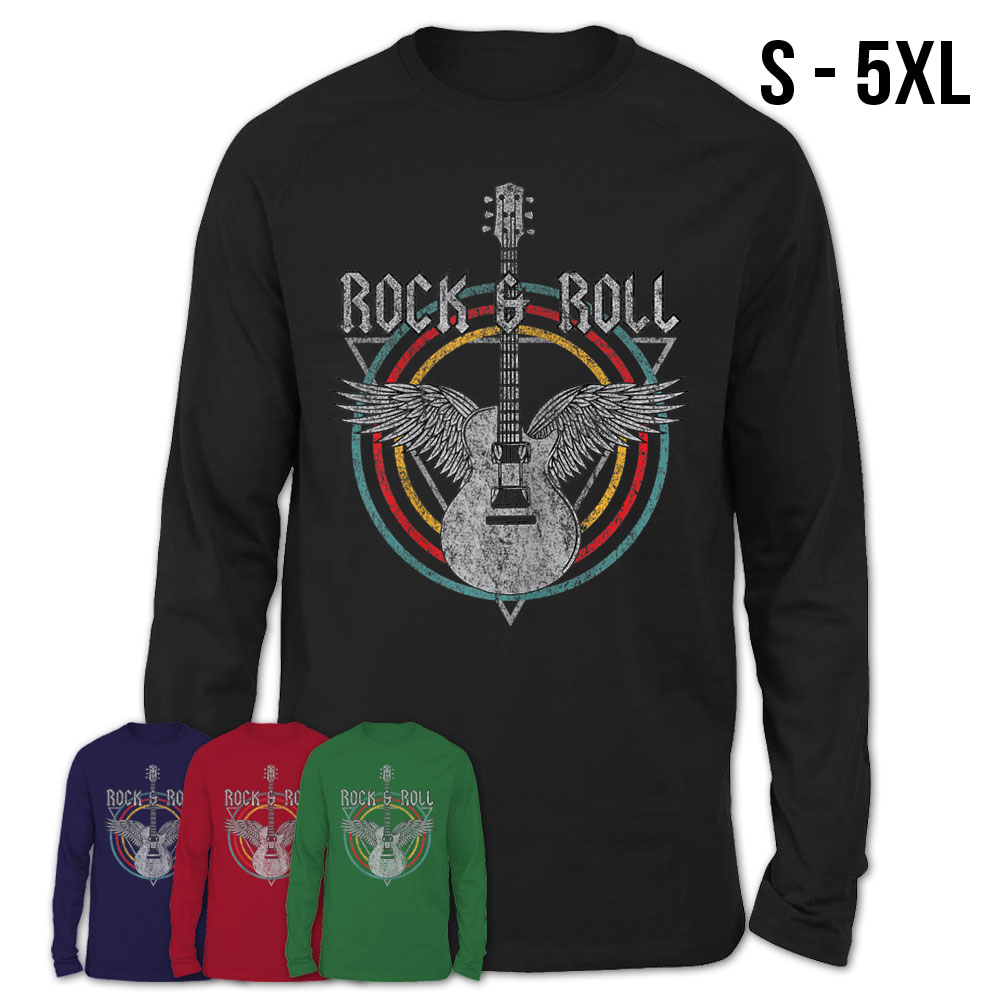The image showcases a stylish long-sleeved t-shirt available in sizes ranging from small to 5XL. The primary shirt, featured prominently in the center, is black with a rounded neck. Its standout design includes a silver guitar with wings, accompanied by the words "Rock and Roll" also in silver. Surrounding the guitar are concentric circles in blue, red, and yellow, adding a vibrant touch to the overall look. The shirt boasts well-crafted cuffs at the sleeves and a neatly squared, loose bottom hem. Additionally, the bottom of the image displays the same t-shirt design in alternative colors: blue, red, and green, offering a variety of choices for buyers.